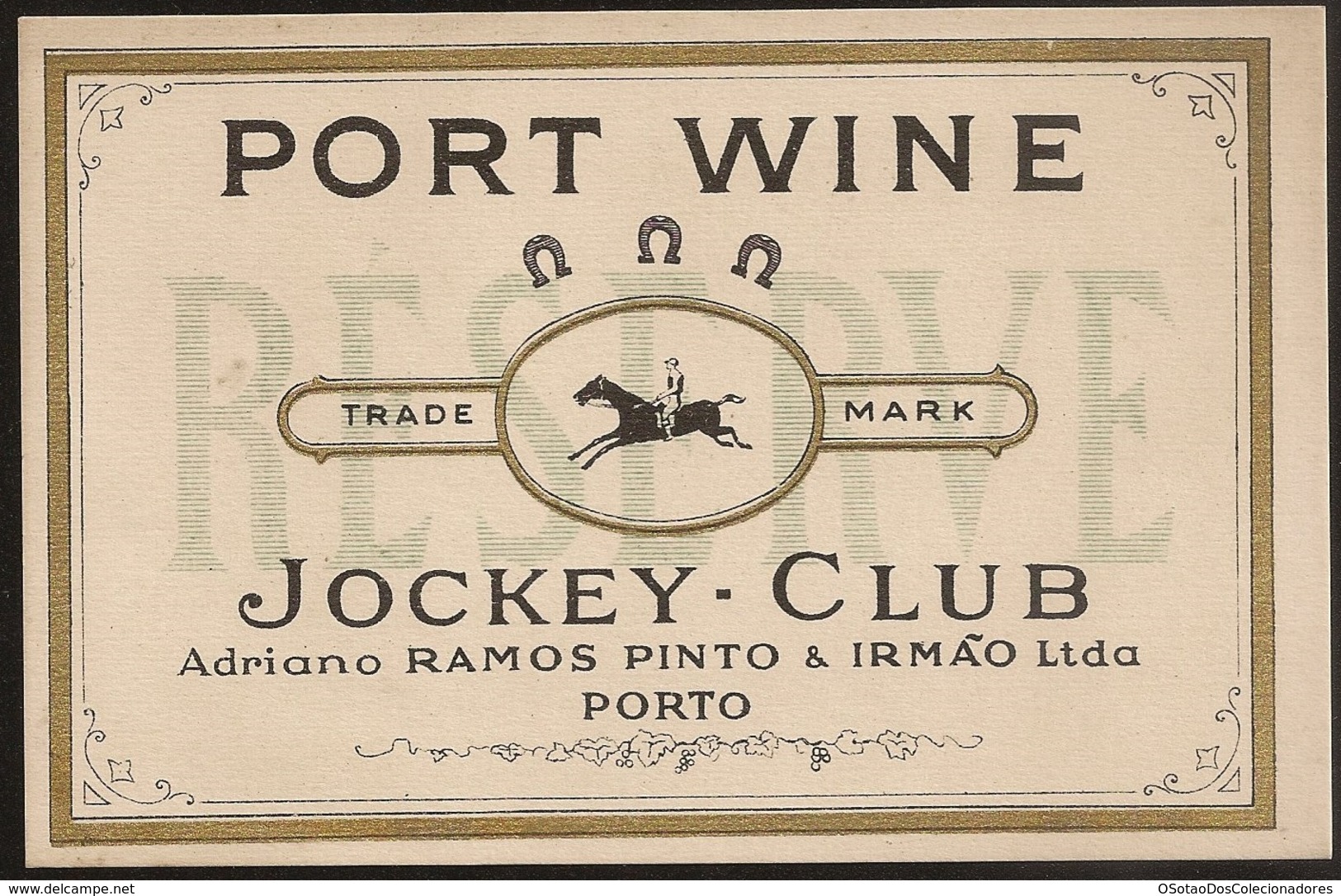The image in question is of a framed wine label with a prominent equestrian theme. The label features a black background and a paper brown frame, giving it a classic, elegant appearance. In the center of the label, set against a light pink backdrop, is a detailed illustration of a black horse in motion with a jockey in full uniform, including a helmet, riding atop. The horse's two front legs are extended lower than the raised back legs, indicating a gallop. Surrounding the illustration is a gold oblong shape. Flanking the image, the word "trade" is inscribed on the left, and "mark" on the right. 

Above this central illustration, the text "Port Wine" is written in black, with three upside-down horseshoes set around the label's logo. Below the illustration, the label reads "Jockey Club, Adriano Ramos Pinto & Irmão Ltda, Porto," also in black text. Additionally, near the bottom corners, there are some ornate designs enhancing the label's aesthetic. Lastly, at the bottom left corner, the website "www.deokam.net" is indicated, while the bottom right corner bears additional unspecified text. The primary colors featured in this composition are varying shades of brown, black, and light pink, blending together to convey a vintage, sophisticated feel, emblematic of the historical brand identity of the product.